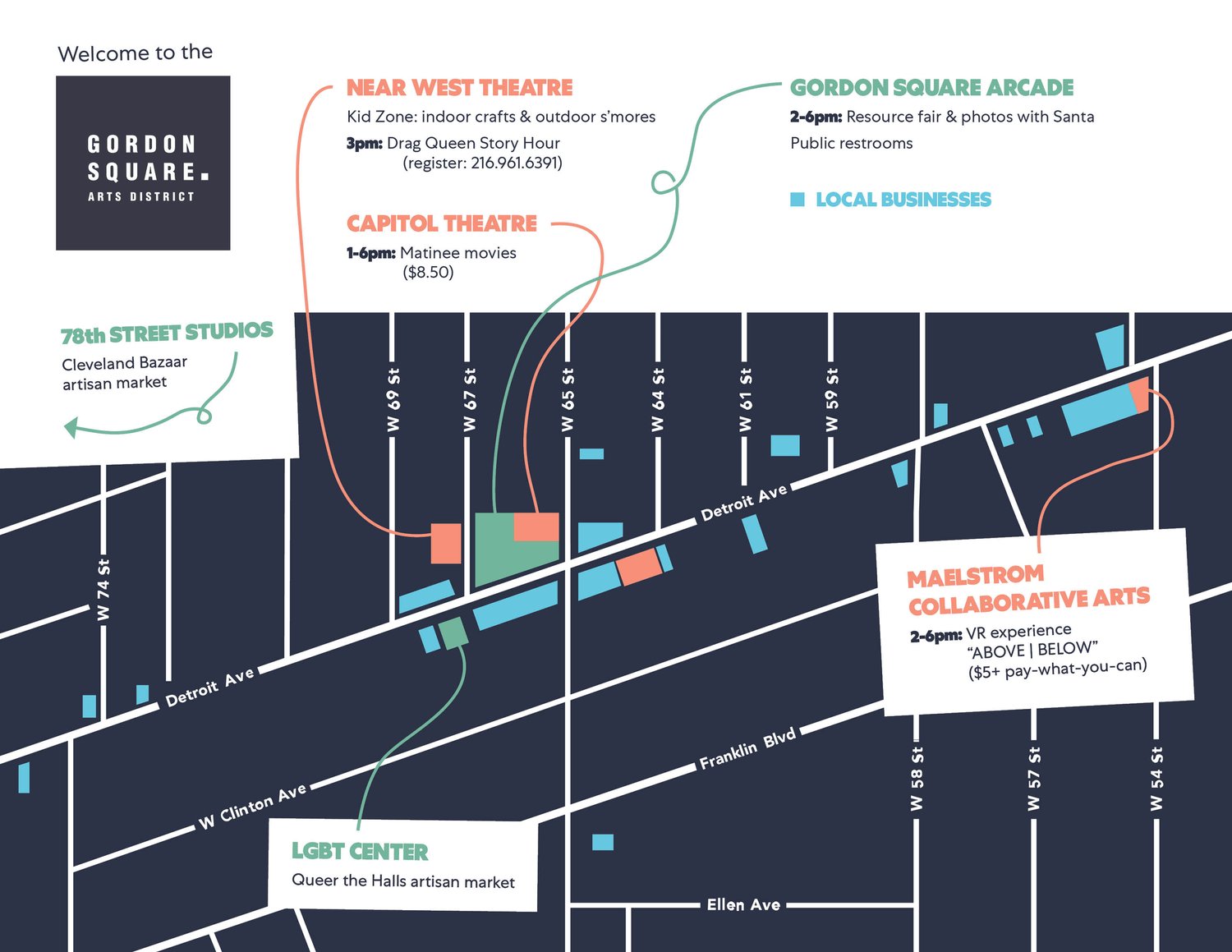This image is a detailed map of the Gordon Square Arts District, featuring a welcoming message in the top left corner that reads, "Welcome to Gordon Square Arts District." The map has a black background with white streets highlighted, including Detroit Avenue, West Clinton Avenue, Franklin Boulevard, and Ellen Avenue, stretching from 54th to 74th streets. Key locations are marked using blocks or triangles in vibrant colors: blues, greens, and oranges. 

Prominent places indicated on the map include 78th Street Studios, the LGBT Center, Maelstrom Collaborative Arts, Near West Theater, Capitol Theater, and Gordon Square Arcade. Additionally, the map designates green for 78th Street Studios, Cleveland Bazaar Artisan Market, Gordon Square Arcade, and the LGBT Center; orange for Near West Theater, Capitol Theater, and Malmstrom Collaborative Arts; and blue for local businesses.

Event features such as a KidZone with indoor crafts and outdoor s'mores, Drag Queen Story Hour, matinee movies, a Resource Fair, Photos with Santa, public restrooms, and the Queer the Halls Artisan Market are also noted on the map. The simplicity of the map, with its reliance on shapes and color codes, provides a clear and organized guide to the district's highlights.